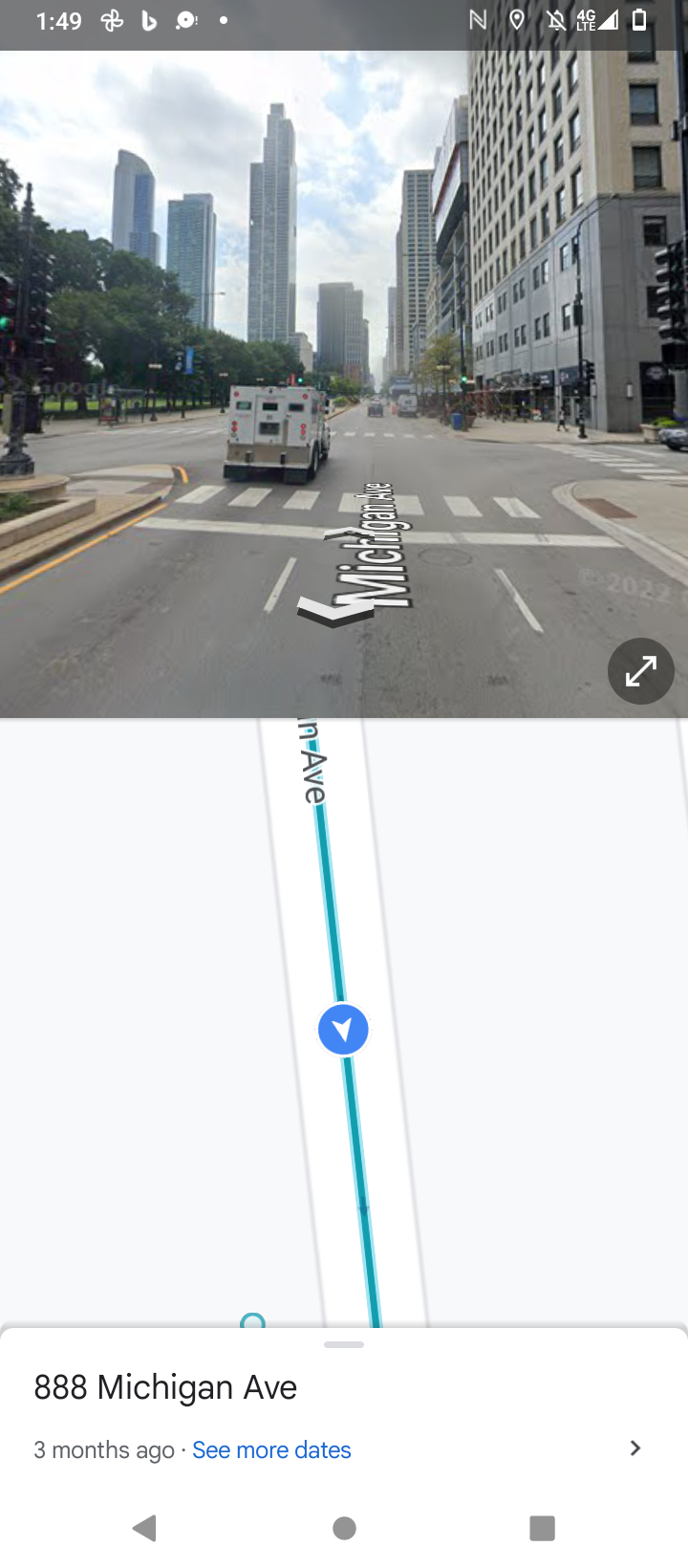This detailed caption is for an image representing a mapping application's screen capture taken on a mobile phone:

The screen grab from a mobile phone's mapping application showcases a detailed map with a highlighted route leading to the location 888 Michigan Avenue, shown in the user's location history from three months ago. The upper half of the screen features an overlaid photograph, providing a real-world view from that very spot on Michigan Avenue. In this photo, we observe a bustling urban scene characterized by numerous tall buildings and green trees lining the left side of the street. A lamppost with its light is also visible on the left. In the driving lane perspective, the middle lane is occupied by a vehicle, while an armored truck can be seen navigating the left lane. The interface allows for navigation through the photograph to the left or right and the option to view it in full screen.